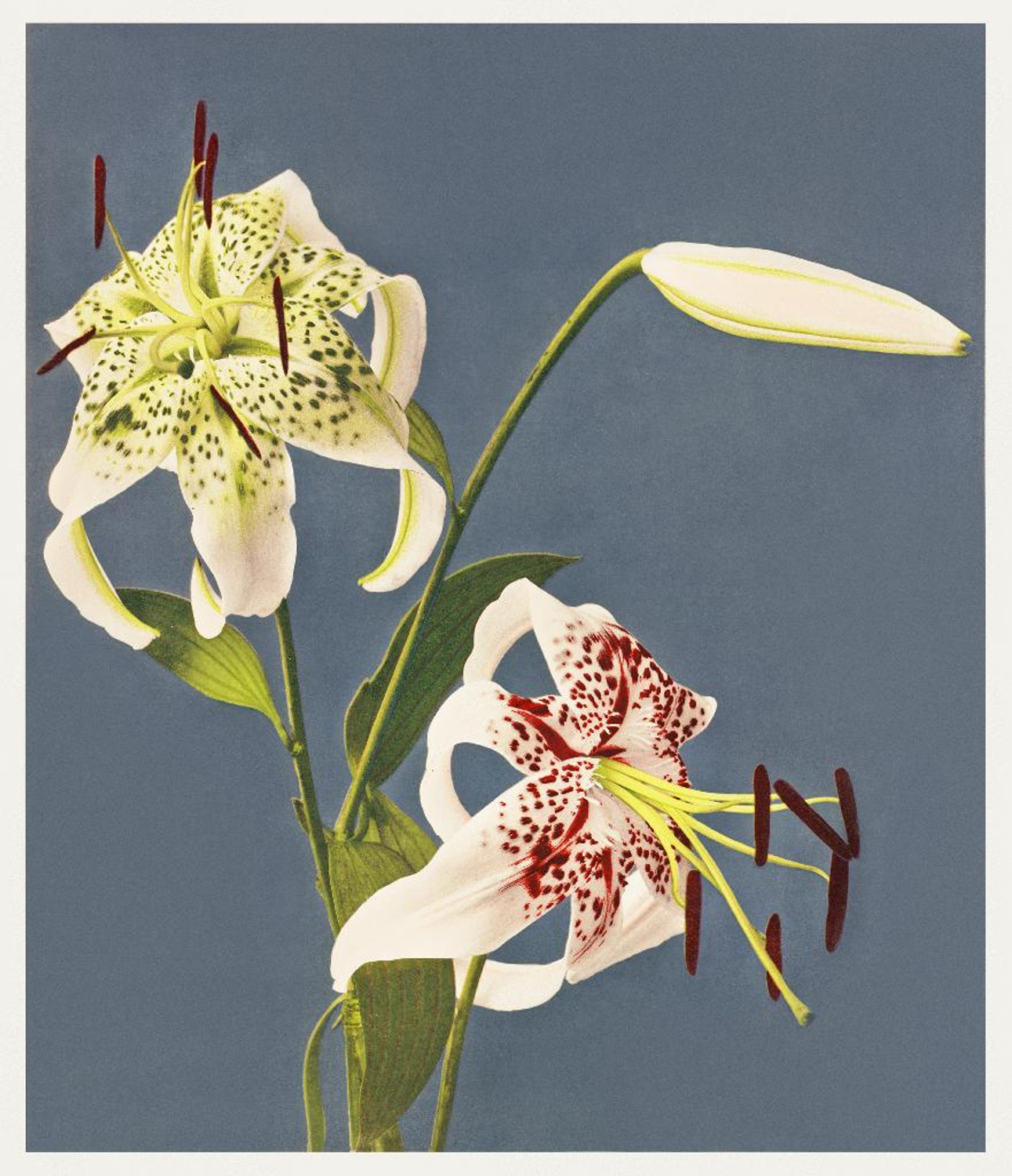This close-up painting features a vividly detailed green plant against a solid blue-gray background. The plant showcases three flowers arranged with two on the sides and one in the middle. The flowers on the sides are open and predominantly white, with the right flower displaying striking red patterns on its petals and the left flower adorned with green patterns. Both open flowers exhibit green antler-like extensions protruding from their centers, with red chain-like seeds dangling from these antlers. The middle flower remains a closed white bud. Additionally, the plant includes distinct leaves; three are easily visible, exhibiting striped patterns from top to bottom, while the fourth leaf discreetly hides behind the right flower and leaf.